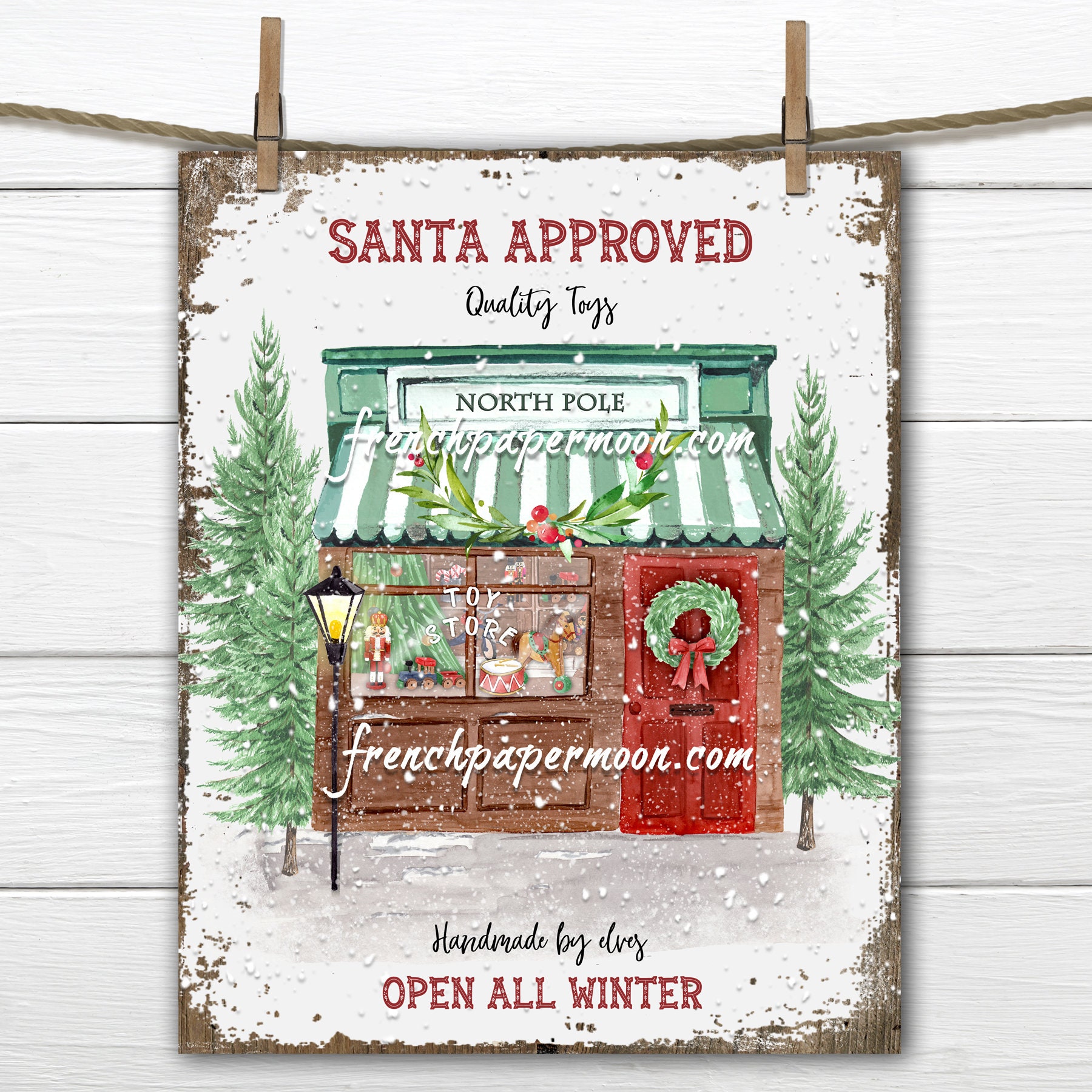The image features a distressed wood sign hanging from a rope with clothespins against a white panel background, giving it a nostalgic, retro vibe. The sign is adorned with falling snowflakes, adding a festive touch. At the top, the headline "Santa Approved" is prominently written in red with "Quality Toys" in small black script beneath it. The centerpiece of the image is an old-fashioned toy shop with a green and white striped awning reading "North Pole". The facade of the shop includes a red door adorned with a Christmas wreath, flanked by pine trees and an old-fashioned light post. At the bottom of the sign, the red text reads "Open All Winter", complemented by the small black script "Handmade by Doug". There are watermarks throughout the image that say "FrenchPaperMoon.com", indicating the ownership of the image.